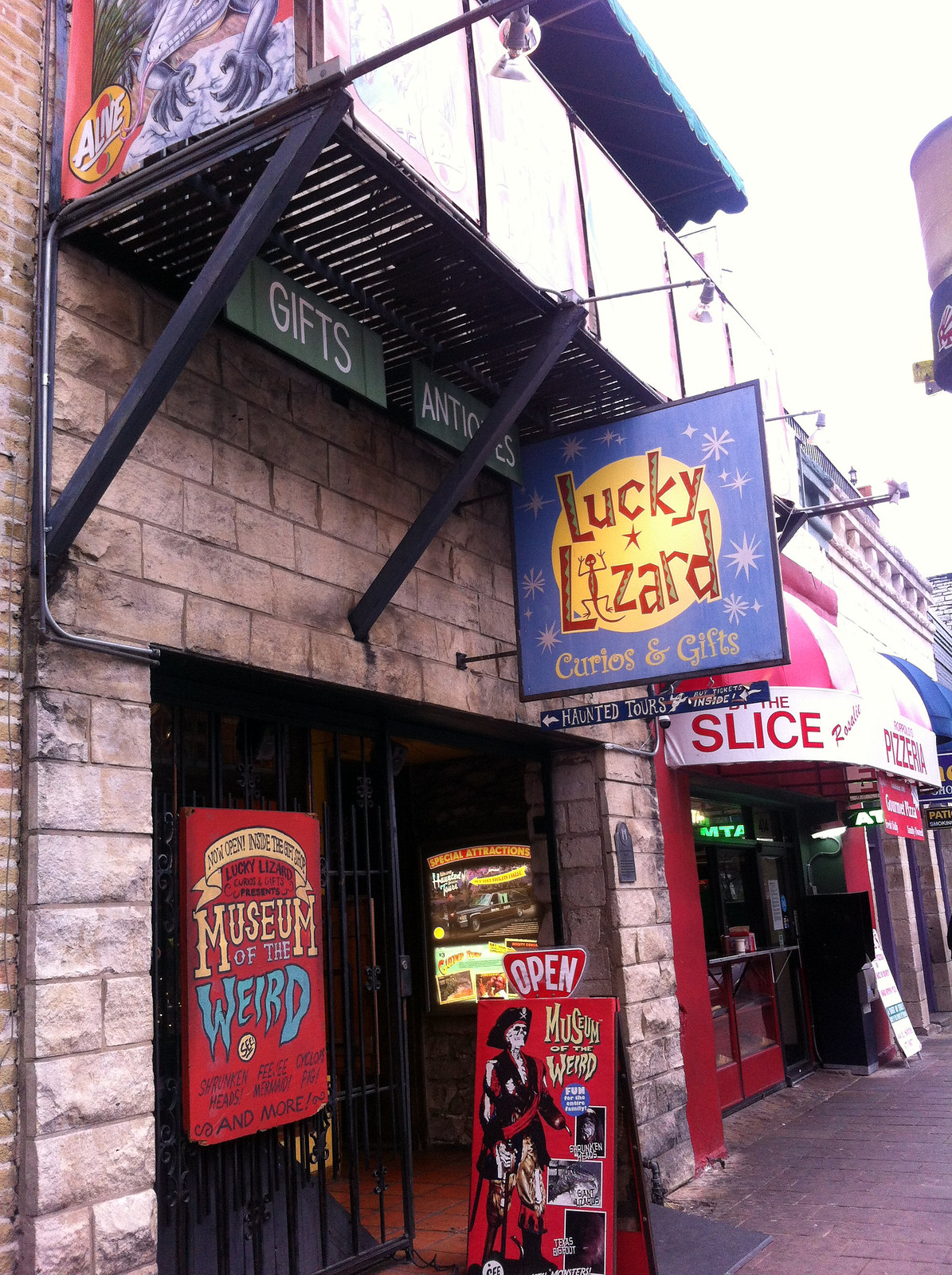The image captures the detailed and vibrant storefront of "Lucky Lizard" gift store. Above its granite-fronted entrance is a prominent blue sign featuring a yellow circle with the store's name "Lucky Lizard" emblazoned in bold red letters. Below, a smaller addition to the sign reads "Curios and Gifts," accompanied by a note that mentions "Haunted Tours Inside." Secured to the store's entrance gate is a red plaque with yellow and blue lettering, announcing "Lucky Lizard, Curios, and Gifts presents the Museum of the Weird." 

In front of the entrance, an A-frame sign displays the word "Open" and images of various unique items available inside the store, including a skeleton pirate illustration pitch for the museum. Above the main signage, extending under what looks like a fire escape, smaller signs indicate "Gifts" and "Antiques." 

Next to the Lucky Lizard, down the street, there is another establishment, likely a pizzeria, identifiable by its red lettering under a white awning that reads "slice." The entire image fades into the street, suggesting the presence of more shops lining the same side as the Lucky Lizard store.